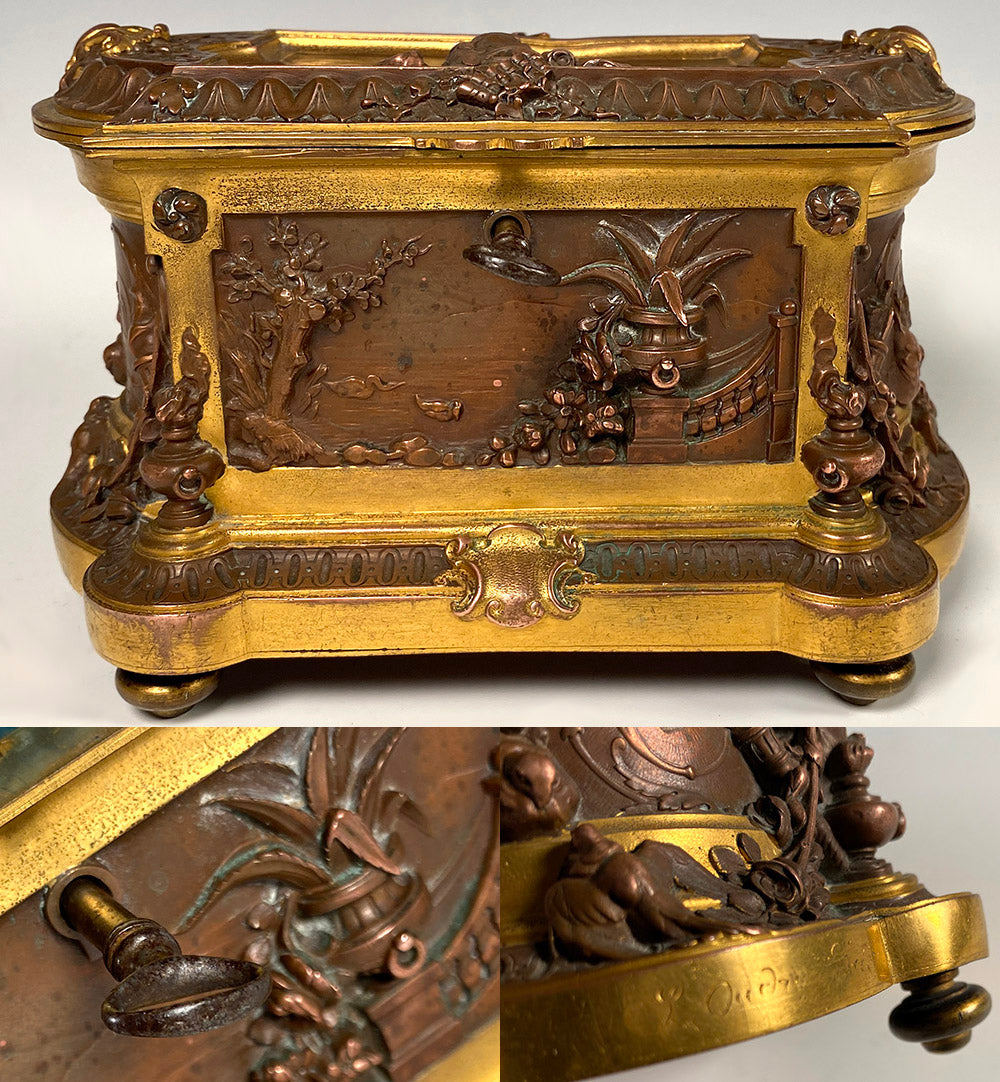The image features an antique wooden storage or jewelry box with a dark brown finish, embellished with gold-colored accents and detailed carvings. This wooden box is likely crafted from quality wood and features intricate brass-like etchings or carvings at the base. The photograph is a collage of three images: the top image displays the entire horizontally-placed box against a gray background, while the bottom two images showcase close-ups of the box's details. The left close-up reveals a detailed carving of a potted plant with large leaves, and the right close-up shows the brass base adorned with an inscription or engraving. Additionally, the corners of the box feature small wooden statues resembling faces or pots. The box appears to be two feet tall and equally wide, with ornate elements, including what looks like a circular peg, possibly for adjusting or securing the box.